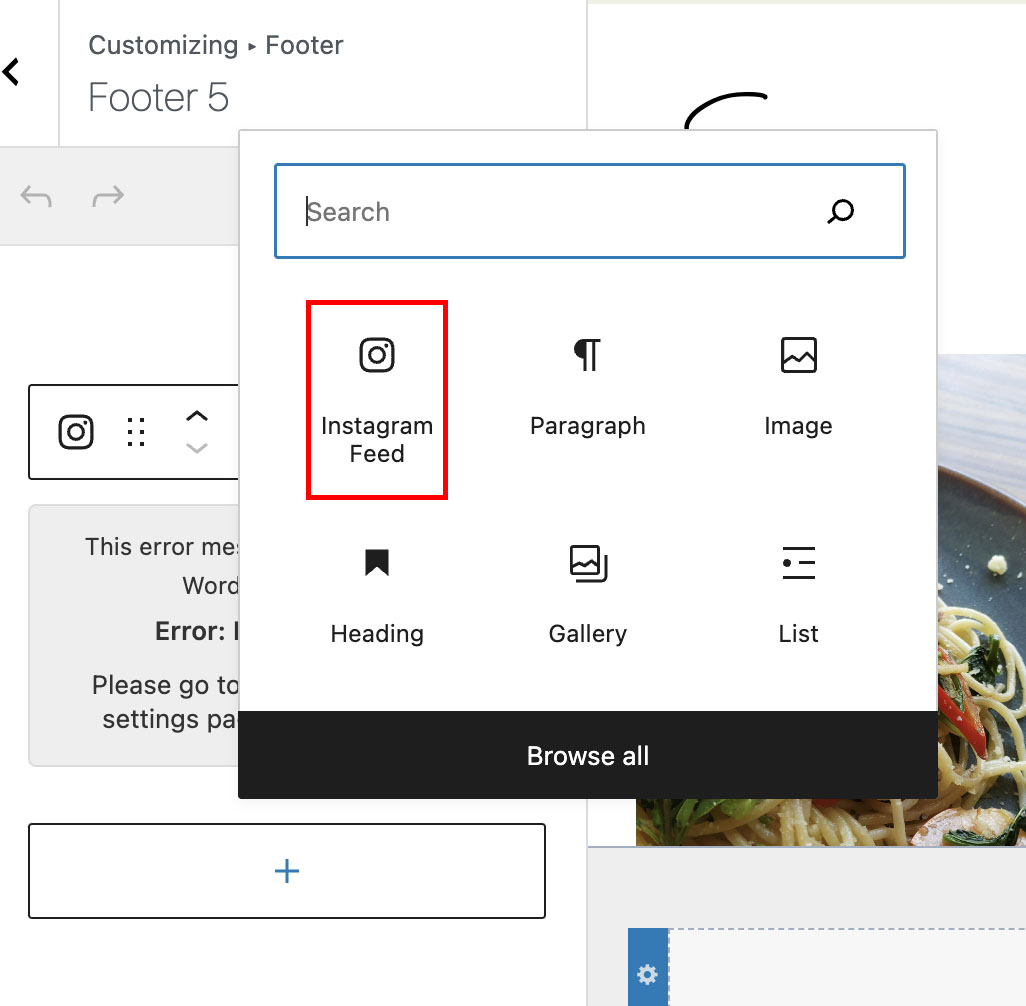This Instagram screenshot captures a multifaceted interface involving a culinary image and various on-screen elements. Central to the image is a dish of cooked noodles, garnished with vibrant peppers and fresh spinach, beautifully plated and set on a table. 

At the top of the screen, there is a customizable footer labeled as "Footer Five." The right side of the image depicts the plate on a table, underneath which a dotted line extends towards the center, intersecting with a wheel-spoke icon and a blue rectangle.

On the left side of the screen, a long rectangular box with a plus sign is visible. Behind and partially obscured by this box, there is an error message reading, "Error. Please go to settings," although much of this gray box's content is cut off.

A search tab box with a blue outline overlays the screen, beneath which icons representing various Instagram post elements are aligned vertically. These icons include:
- Instagram feed with a camera icon.
- Paragraph with a paragraph symbol.
- Image represented by a square featuring a stylized mountain range.
- Heading denoted by a black square with a triangular bottom cut-out.
- Gallery, shown as a mountain icon within a square, accompanied by an additional line outside it on the right.
- List symbolized by three lines, with the second line starting with a dot.

Below these icons, a "Browse All" label is displayed in white text against a black background.